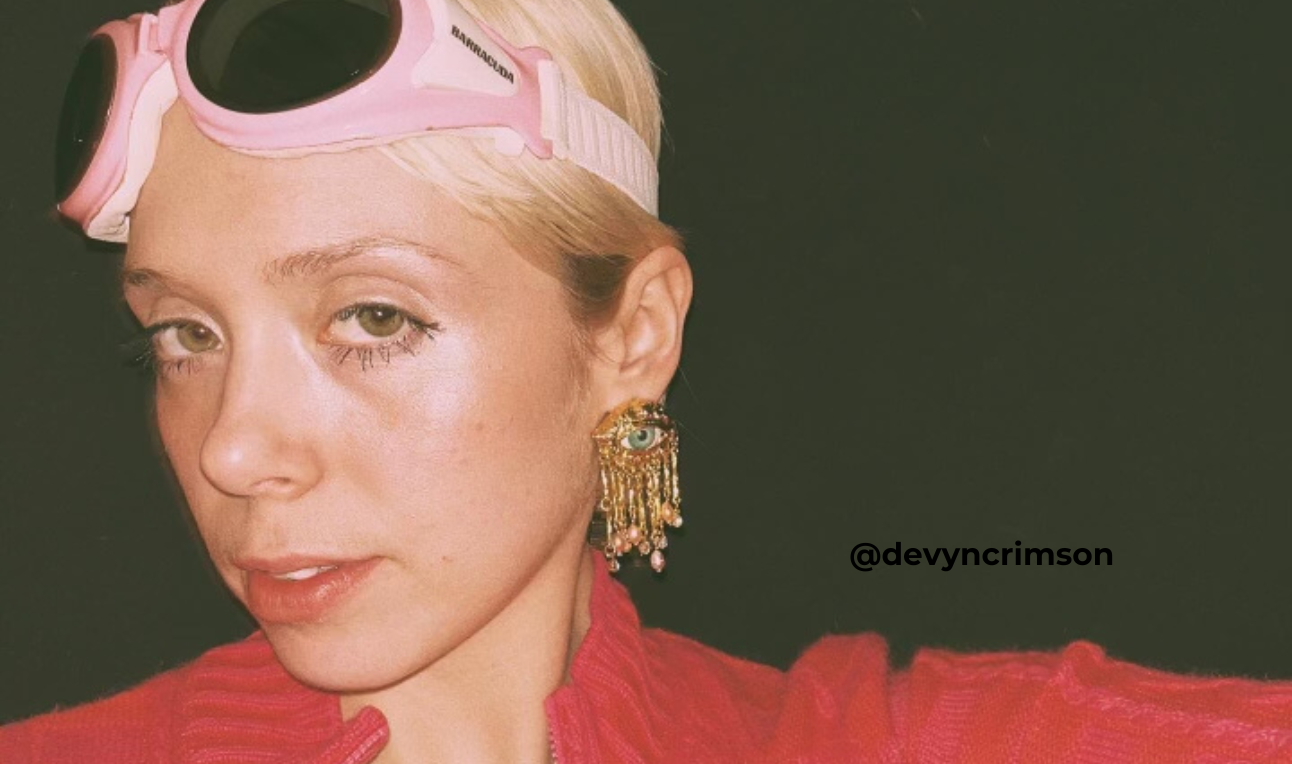The image features a young Caucasian woman with a platinum blonde, short hairstyle that transitions into darker tones further down. She has a light complexion with slight bags under her green eyes and ruby red lips. On her forehead sits a pair of pink swimming goggles branded with "Barracuda." She wears an elaborate earring in her left ear, which is fully visible as she is turned towards the right. The earring features a striking blue eye with a black pupil at the center, surrounded by gold, and adorned with gold chains and pink beads dangling from it. Her makeup is minimal, with a hint of lumpy mascara. She is dressed in a red top, characterized by many folds and creases, which appears to have a zip or fastening in the front. The photograph has a Polaroid aesthetic against a matte dark gray background, and at the bottom right, it is labeled with the Instagram handle "Devin Crimson." Her expression is subtle, almost a small smile, but she also seems somewhat tired.